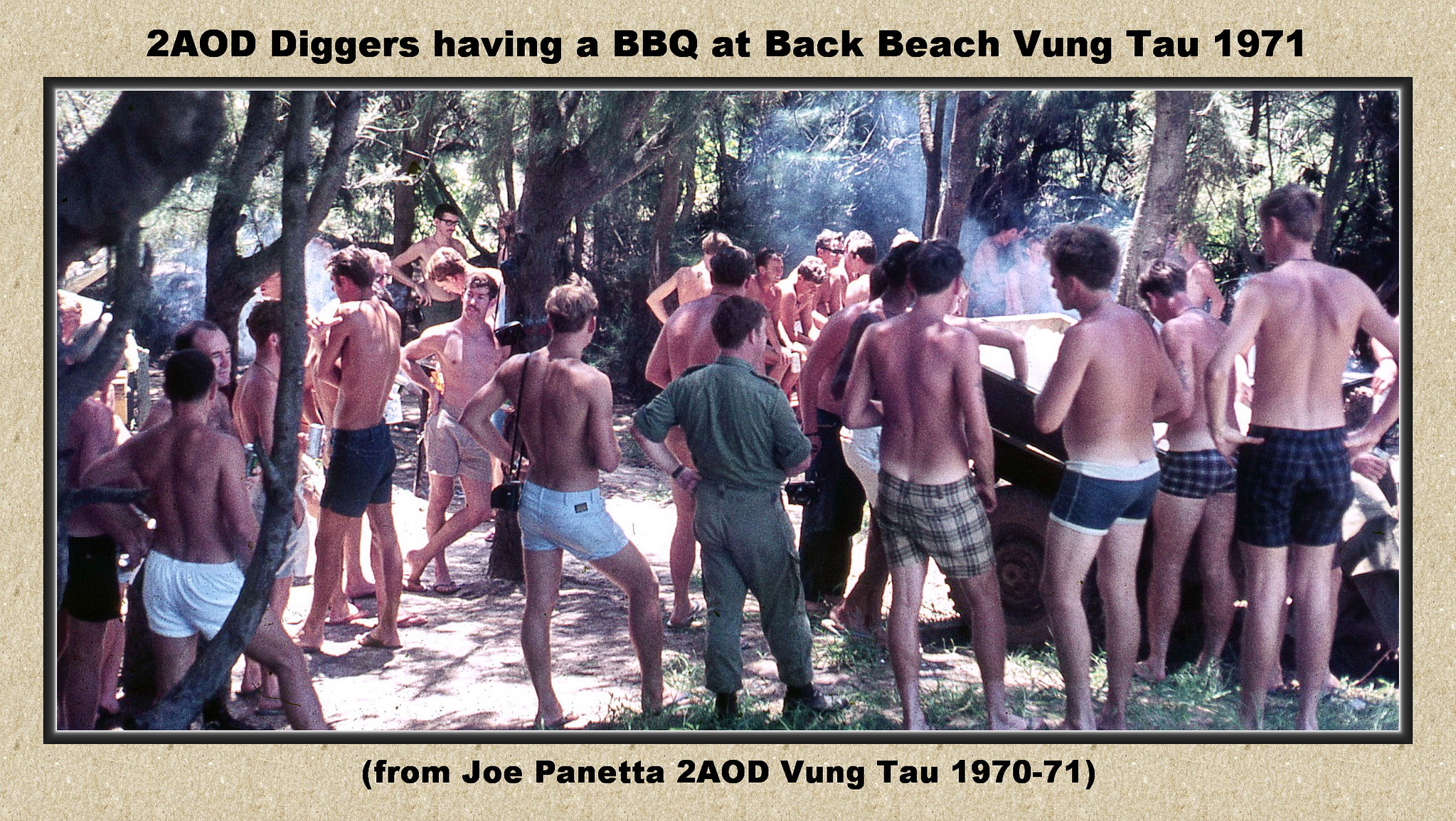The photograph depicts a group of young men, likely around 17 years old, standing in a forested area, surrounded by trees, grass, and natural debris. Most of the boys are shirtless and wearing only shorts, boasting tanned backs indicative of significant time spent outdoors. Among them, one man stands out fully dressed in a dark green button-down collared shirt, matching pants, and black boots, likely a leader or supervisor. A barbecue is in progress, and there's a truck or cart nearby emitting smoke. The image is framed with a light brown border, with an inscription at the top reading, "2 AOD diggers having a barbecue at Back Beach, Vung Tau, 1971." At the bottom, the border notes, "From Joe Panetta, 2 AOD, Vung Tau, 1970-71."